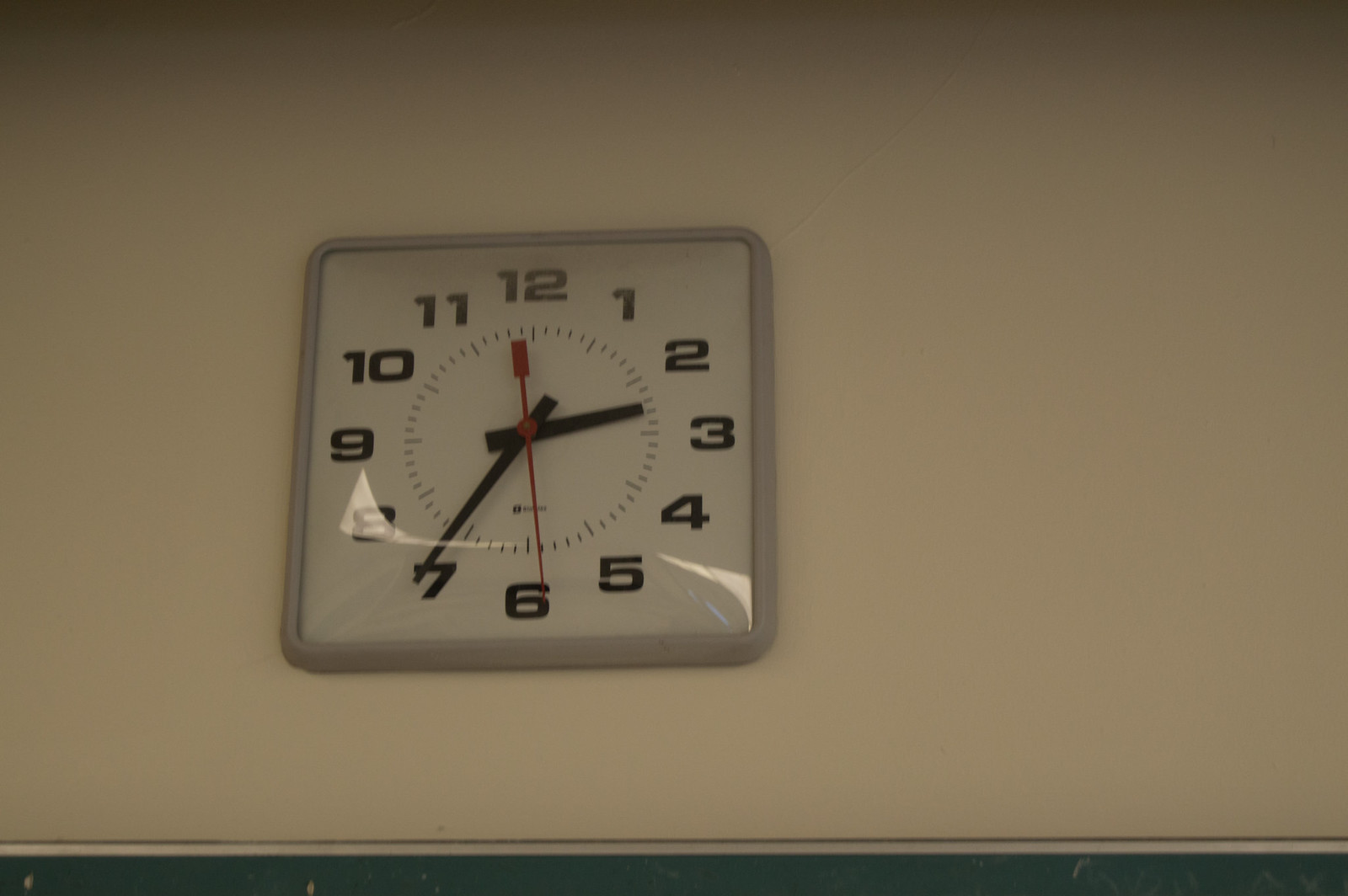The photograph showcases a square-shaped wall clock with a gray plastic body and a clear plastic cover, mounted at the center of a predominantly white wall with a green strip running horizontally at the bottom. The clock face is white, featuring large, bold black numbers from 1 to 12, with four small black lines between each number to mark the minutes. The hour and minute hands are solid black, while the second hand is red. The clock indicates the time is 2:36 and 29 seconds. Above the 6 o'clock position, there is a manufacturer's name that is too small to be legible. The image is captured from a slightly lower angle, adding perspective to the clean, simple design of the clock against the contrasting backdrop.